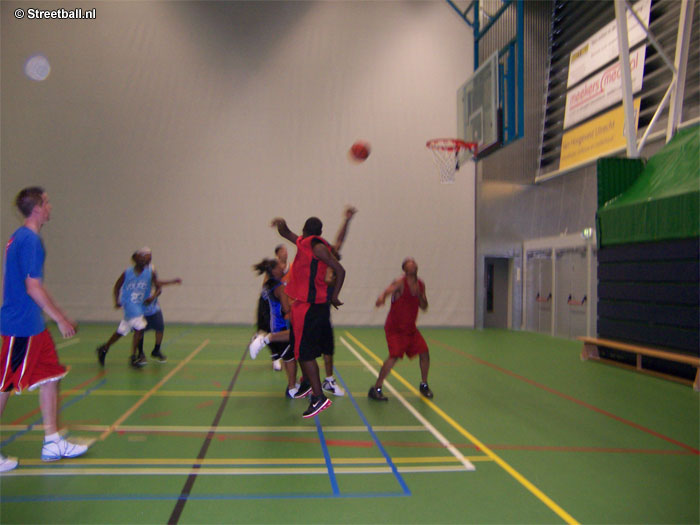The image depicts an in-motion shot of a basketball game being played indoors, possibly at a recreational center or school gymnasium. The photo, slightly blurred due to the motion, captures eight gentlemen actively engaged in the game on a green court marked with various colored lines—yellow, blue, red, black, and white—indicative of a multi-purpose facility. At the top left corner, the photo bears the text "streetball.ni" alongside a blue glare mark from the camera. To the left, a player donning red basketball shorts and a blue shirt is seen looking to the right, while another player in red and black shorts and a red shirt is captured in mid-air, having just shot the ball toward the hoop located on the right side of the image. The players' jerseys range from blue to red, and there’s a notable presence of different colored shorts. The backdrop includes a white multi-storied wall with several large entrance doors to the gymnasium on the right side, above which three signs can be seen—two white and one yellow. Additionally, there are closed off black and green bleachers beside these doors and a long, empty wooden bench on the right-hand side of the court.